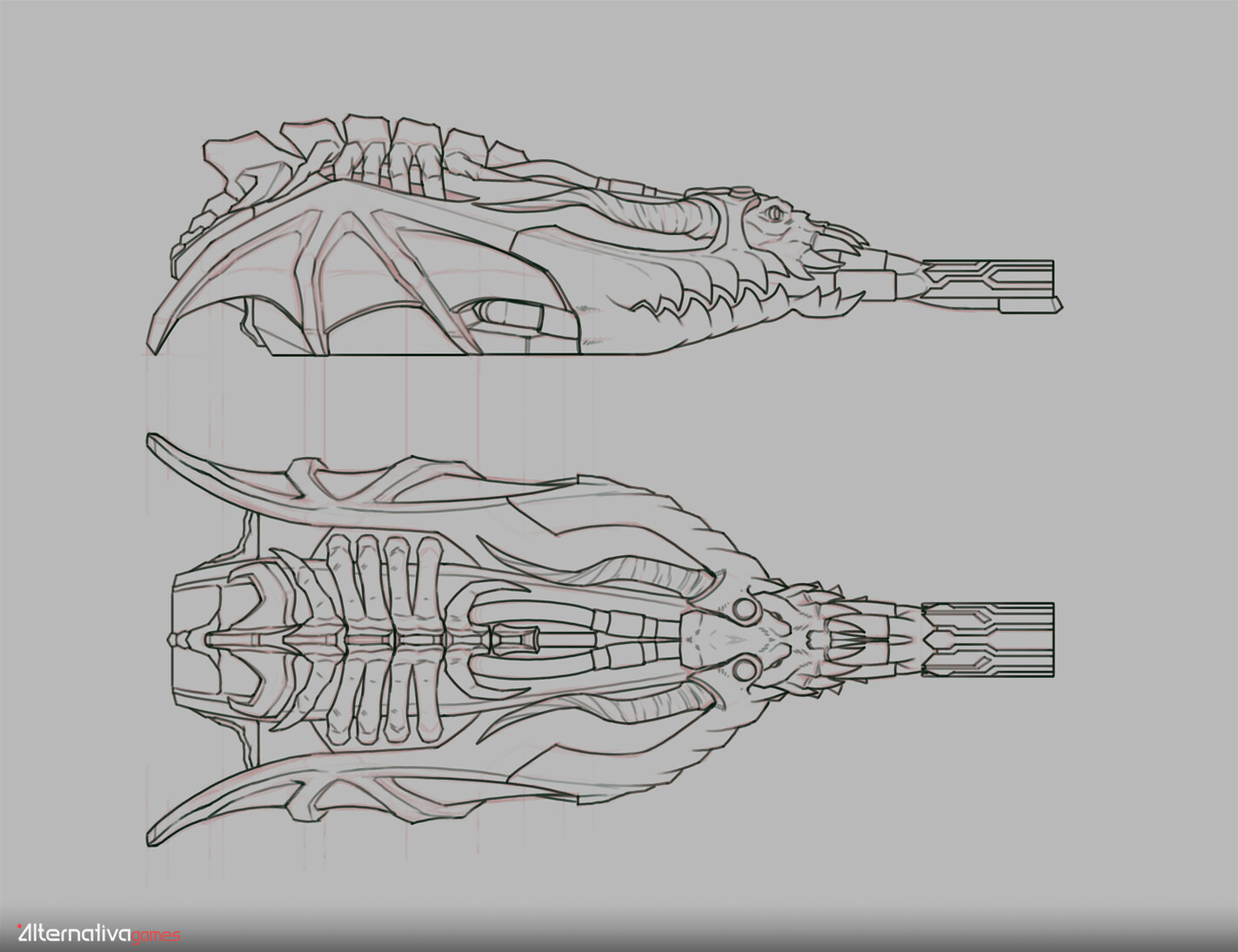This black and white illustration, likely from a game cover titled "Alternativa," showcases a highly detailed, alien-like skeletal figure. The drawing is bifurcated into two views: a side view at the top and an aerial view at the bottom. Dominating the scene are intricate black line details with subtle touches of red outlining certain elements. The figure appears to have a complex vertebrae structure and a prominent, elongated nose or beak-like extension. The side view reveals large teeth and a mouth, suggesting a creature rather than a machine, while the overhead depiction emphasizes its wings, horns, and what appears to be a cloak, lending it a tribal or ethereal quality. The whole composition is cast against a gray background, enhancing the contrast and intricacy of the creature's design.